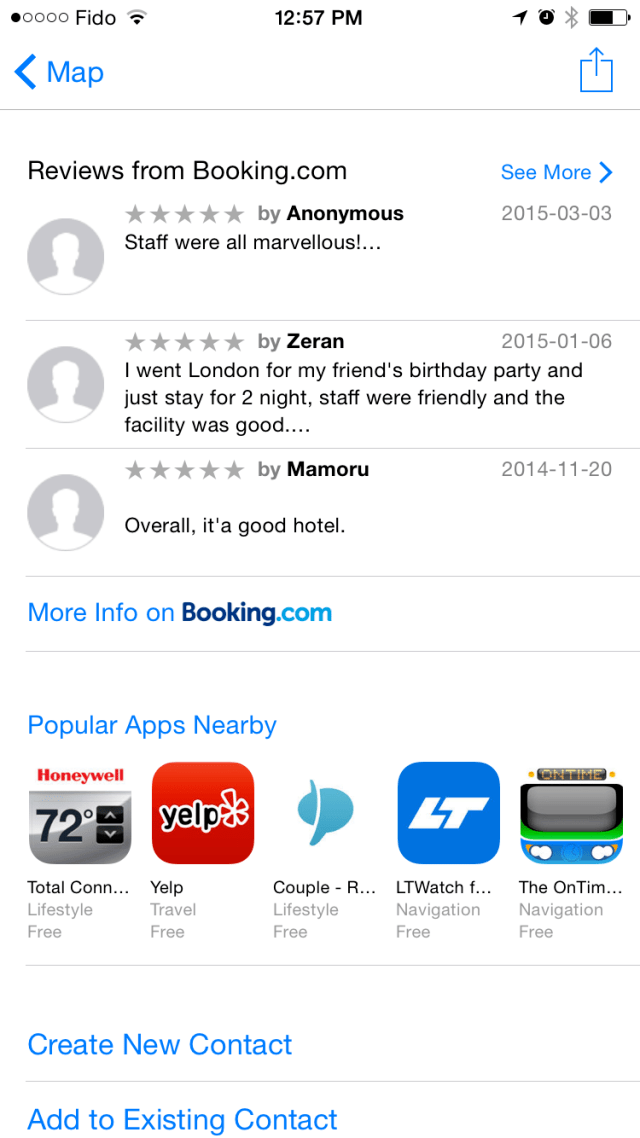This is a detailed screen capture from the App Store on an iPhone, displaying a specific app page with various UI elements and user reviews. 

At the top of the screen, a rating indicator shows one out of five dots highlighted next to the app name, "Fido." The status bar displays the time as 12:57 PM, along with a Wi-Fi signal indicator (two out of three bars lit), location icon, alarm clock icon, Bluetooth icon, and a battery icon showing approximately 75% charge.

Below the status bar, there is a navigation section featuring a blue "Map" icon with a back button, and a blue download icon. This section is followed by a reviews section titled "Reviews from Booking.com" with a "See more" link in blue text.

Three user reviews are listed:
1. **Anonymous** (5 stars, dated 2015-03-03): "Staff were all marvelous."
2. **Xeron** (5 stars, dated 2015-01-06): "I went to London for my friend's birthday party and just stayed for two nights. Staff were friendly and the facility was good."
3. **Mamoru** (5 stars, dated 2014-11-20): "Overall, it's a good hotel."

Each review is accompanied by a generic profile picture. Below the reviews, there is a hyperlink in blue text labeled "More info on Booking.com."

Further down, there is another blue hyperlink titled "Popular apps nearby," listing adjacent apps such as Honeywell, Yelp, Couple, LT Watch, and The On Time, along with their respective icons.

At the bottom of the screen, two blue hyperlinks offer options for contact management: "Create New Contact" and "Add to Existing Contact."